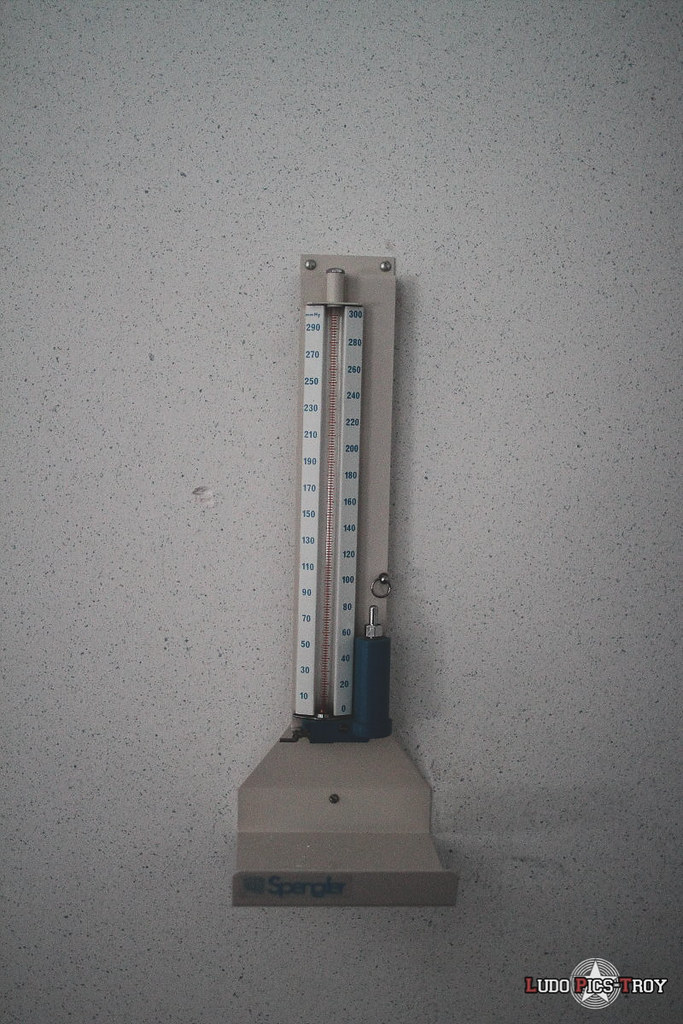The image captures an outdoor thermometer positioned on a white, speckled ledge, possibly made of stucco or plaster. The thermometer, manufactured by SpurPly, features a gray backing and bottom. The temperature is indicated by a red line, with gradations marked on both sides of this line. Adjacent to the numbered section of the thermometer, there's a blue component that appears to be part of the device, with a screw protruding from the top and a nail with a small metal ring on it. The top of the thermometer is fastened together with two screws. The ledge it rests on has a gouged surface, adding texture to the scene. At the bottom of the image, the text "Ludopix Troy" is visible.